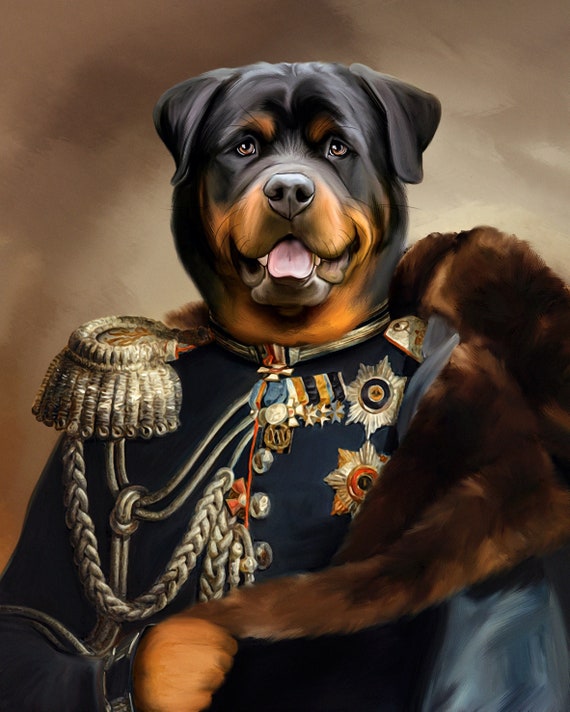This detailed portrait, possibly a computer-generated image or painting, features a large, stereotypical-looking dog with a prominent snout and floppy ears, resembling a Rottweiler. The dog, depicted with a mouth slightly open as if panting, is personified by sitting upright in a dignified pose, wearing an elaborate 18th-century military uniform reminiscent of those worn by Napoleon. The uniform is adorned with various medals, gold ropes, and chains, and it features a fur-lined shoulder. The dog showcases black and brown coloring and emanates a sense of happiness, suggesting it might be receiving an award. The image merges elements of canine and human characteristics, creating a striking blend of a regal military figure and a loyal dog.